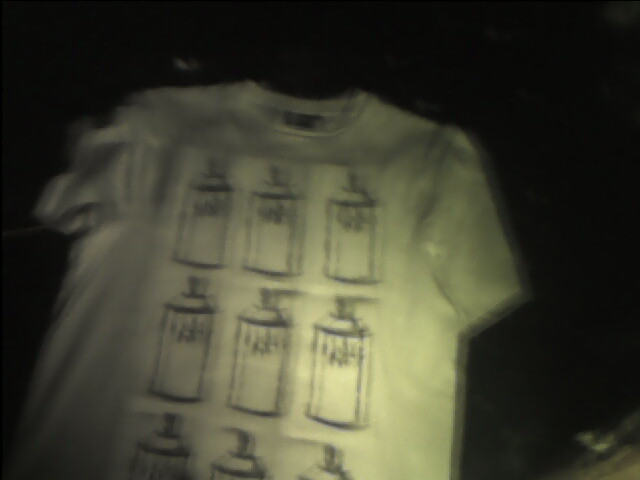In the horizontally elongated, rectangular photograph before me, the image presents an extremely blurry and darkened visual, dominated by a black background with a slightly lighter streak in the lower right corner. Amidst this obscured scene, a lighter-colored t-shirt, potentially white or beige, with a crew neck and short sleeves, can be discerned. The t-shirt features an illustration, although indistinct and hand-drawn, of nine cans that could be either whipped cream or spray paint. These cans are rendered in black outline, accompanied by scribbled, indistinguishable writing at the top, serving as a label. The overall artwork on the t-shirt lacks professional refinement, contributing to its enigmatic and amateurish appearance.